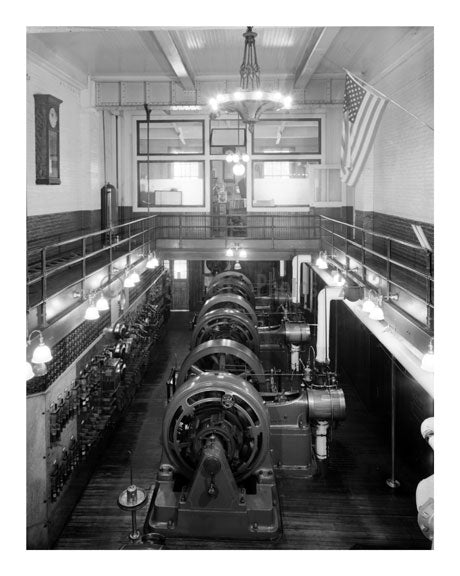This black-and-white photograph captures an industrial setting, most likely a power generation room housing six large machines resembling generators or turbines. These machines have circular coils, indicating their use in generating electricity. The room features a two-floor layout with the machinery centrally positioned on what appears to be a dark hardwood floor. On the bottom floor to the left, an array of control panels, switches, and indicators line the wall beneath a series of lights. Above, a metal railing runs the length of the second floor, from where a wooden grandfather-style clock can be seen affixed to the wall. 

The top third of the walls are white, while the bottom third is constructed of dark, perhaps black or brown, bricks or wood. Hanging lights with multiple bulbs, including a chandelier-like fixture, illuminate the space, despite windows at the far end that suggest daylight outside. The room is punctuated by an American flag displayed on the right wall, adding a patriotic touch. In the background, a series of rectangular windows flanks a central doorframe, enhancing the industrial yet orderly ambiance of the space.